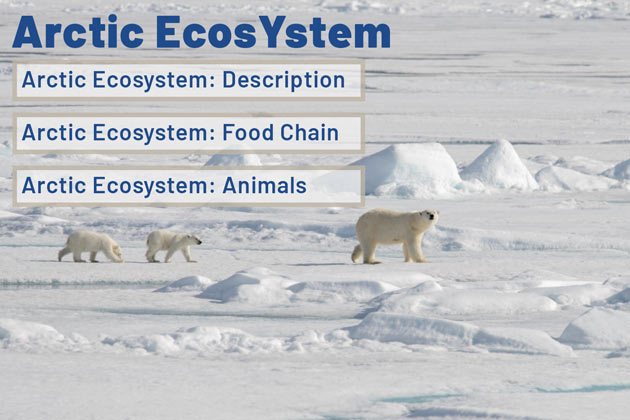The image portrays a vast Arctic ecosystem, characterized by an extensive snow-covered landscape with subtle hills formed by windblown snow. Walking from left to right across this icy expanse are a mother polar bear and her two small cubs, their white fur blending seamlessly with the snowy environment. In the top left-hand corner of the image, dark blue lettering prominently titles the scene as "Arctic Ecosystem," followed by smaller text boxes outlining "Arctic Ecosystem Description," "Arctic Ecosystem Food Chain," and "Arctic Ecosystem Animals." The absence of other animals and landmarks, such as glaciers, emphasizes the stark, cold isolation of their habitat.